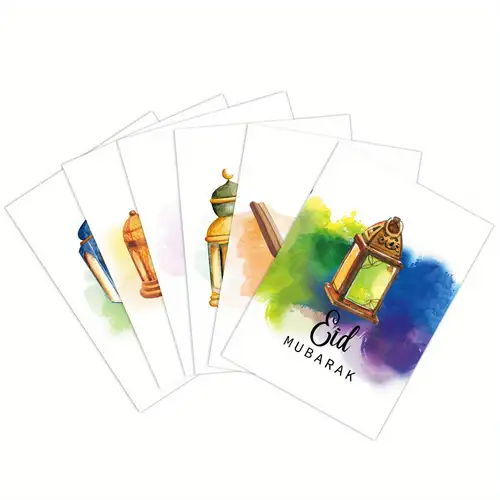This is a digitally created image featuring a set of six rectangular cards, arranged in a semi-circular, fan-like manner. Each card seems to feature a lantern with watercolor-style colors. The rightmost card is fully visible and displays a green lantern with a gold pyramid top, alongside a swirl of blue and green paint. The text "Eid Mubarak" is prominently written on this card, signifying that these cards are designed as a celebratory present for a Muslim viewer celebrating Ramadan. The remaining five cards, slightly hidden behind the foremost one, also appear to depict various lanterns in a similar classic watercolor style. The background of the image is white, further highlighting the vibrant colors and festive theme of the lantern illustrations.